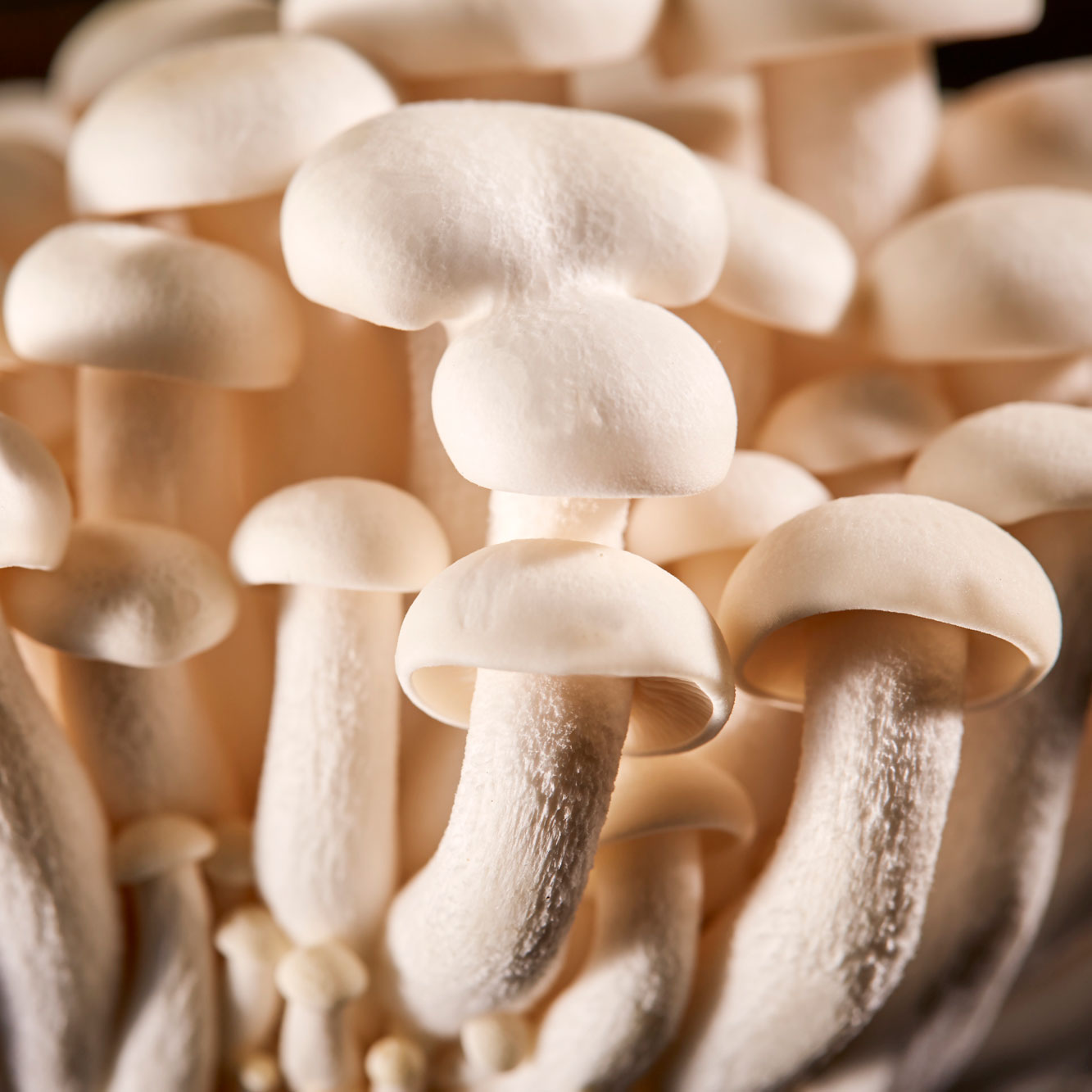This photograph, possibly computer-generated, captures an intricate cluster of predominantly white mushrooms growing together in a seemingly haphazard yet organic formation. The scene is dominated by the off-white, slightly peach-tinged caps set against rougher, hirsute stems. These fungi vary in size, with smaller, fuzzier mushrooms appearing in the lower, slightly out-of-focus portion of the frame, and larger, smoother-capped mushrooms dominating the foreground. Some of the tops are hollow, revealing the delicate gill-like filaments within. The mushrooms appear to grow from a common root, curving upwards as if reaching for light, and the overall arrangement—piled upon each other—suggests a surreal, almost fantastical, quality.